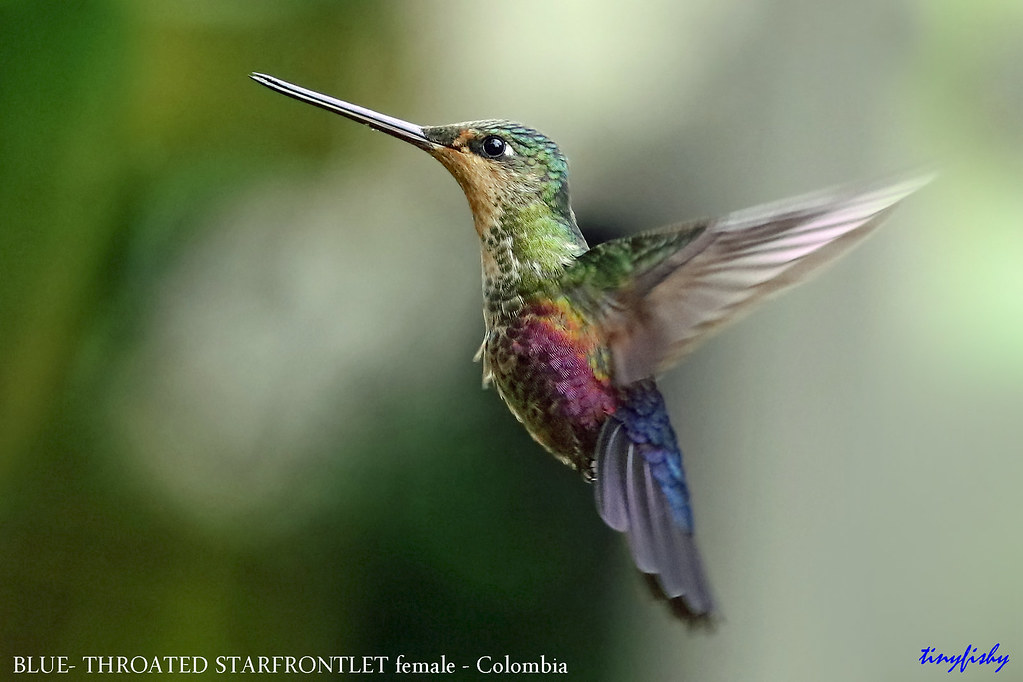A high-resolution, close-up photograph captures a beautifully detailed blue-throated starfrontlet hummingbird, identified as a female from Colombia by text at the bottom left. The bird, seemingly frozen in mid-flight, has a long, silvery beak and is facing left, with one eye appearing to gaze directly at the viewer. The vibrant metallic feathers on its head showcase shades of emerald green and aqua, transitioning into a golden throat. Its wings exhibit hues of green with silvery tips, while the belly contrasts with rich ruby tones accented by yellow and green. The tail feathers are a striking blend of royal blue and purple, ending in silver. The background is blurred in varying shades of green, suggesting the presence of trees, giving the impression of a forest setting. The artist's signature, "Tiny Fisbee," appears in blue script to the right, enhancing the curated, guidebook-like quality of the image. The detailed focus allows for the clear visibility of individual feathers, emphasizing the bird's intricate beauty and motion.